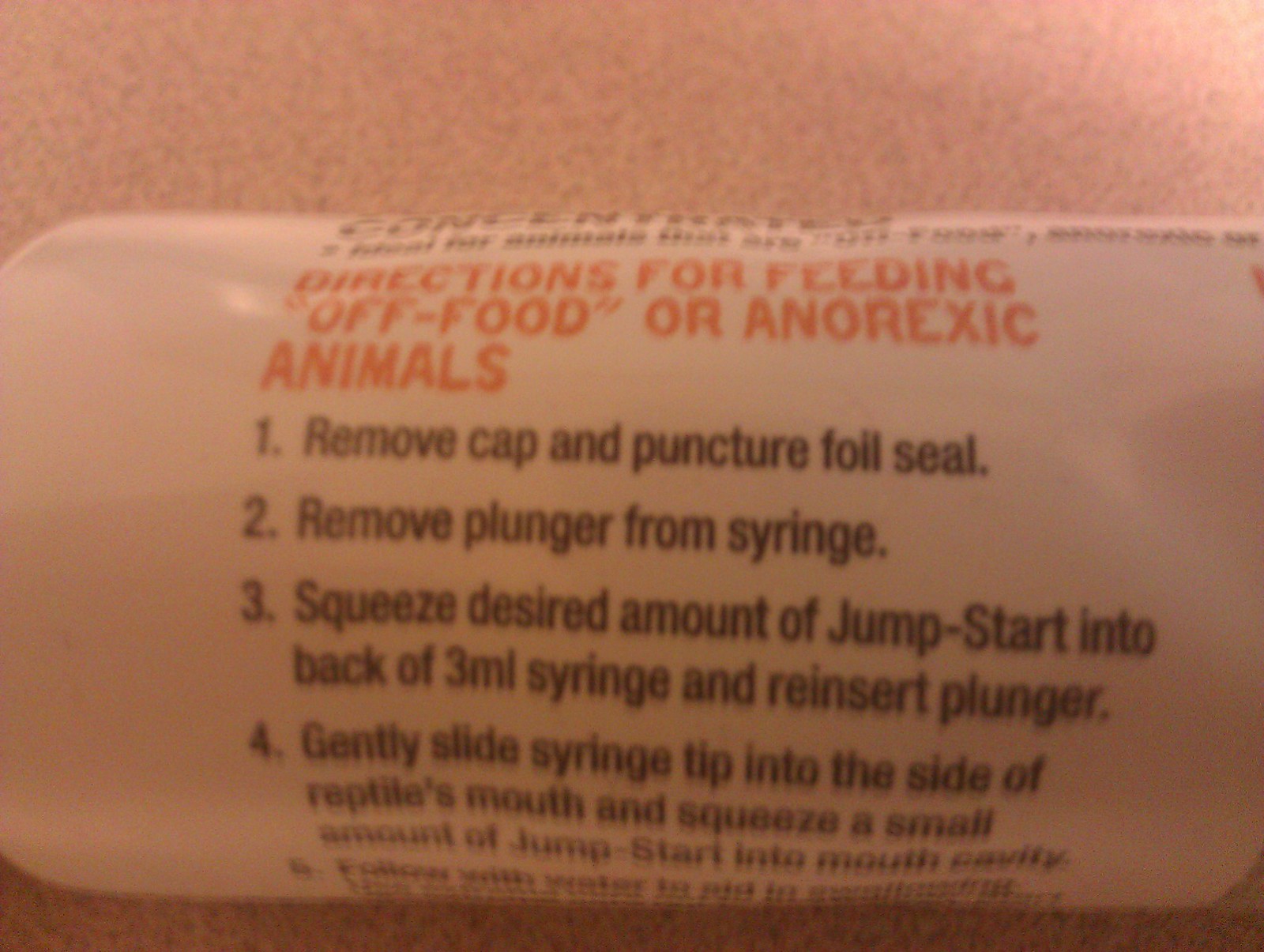The image depicts a slightly blurry, horizontally placed white plastic tube, laying flat on a speckled, pinkish surface, most likely indoors. The text on the tube is a set of step-by-step instructions for administering a product called "Jumpstart" to feeding-off or anorexic animals, particularly reptiles. At the top, bold red capital letters read: "DIRECTIONS FOR FEEDING OFF-FOOD OR ANOREXIC ANIMALS." The instructions below are written in black and detail the following: 

1. Remove the cap and puncture the foil seal.
2. Remove the plunger from the syringe.
3. Squeeze the desired amount of Jumpstart into the back of a 3-milliliter syringe and reinsert the plunger.
4. Gently slide the syringe tip into the side of the reptile's mouth and squeeze a small amount of Jumpstart into the mouth cavity.

The image does not clearly show step five, as it is blurry and cut off. Despite the slight blurriness of the photograph, most of the text is legible.